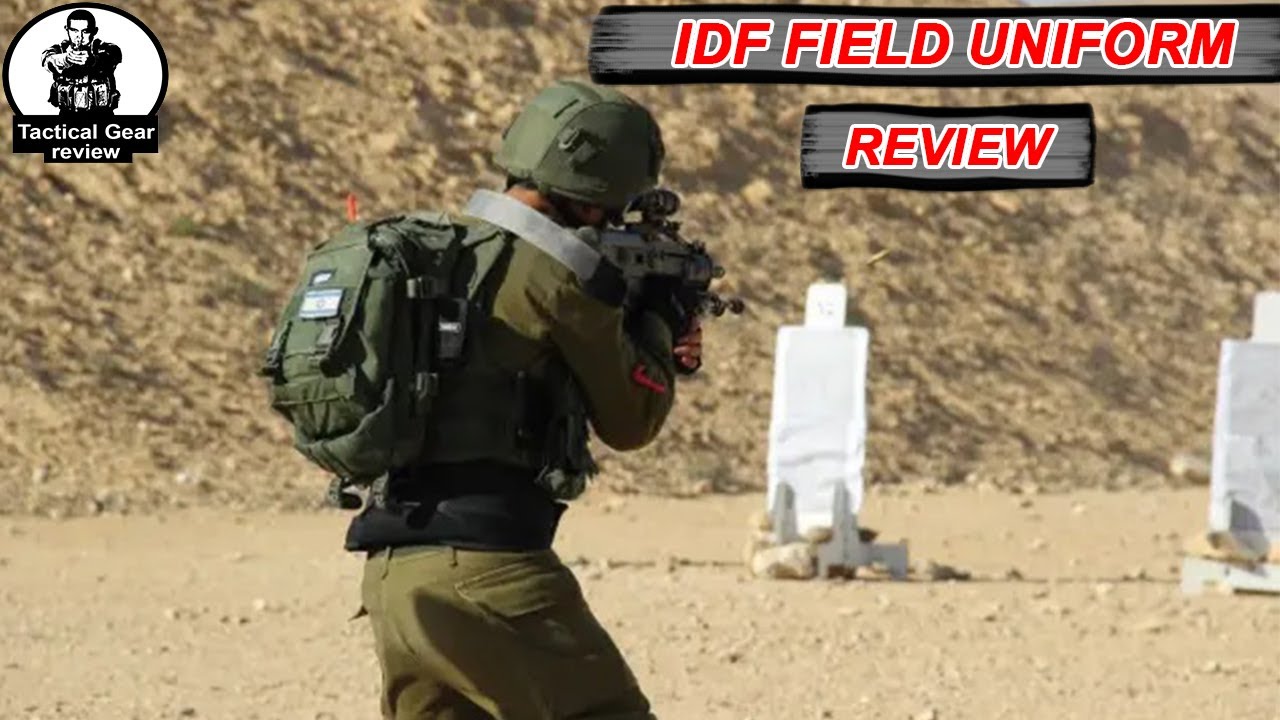The image depicts a soldier or tactical enthusiast from behind, centrally positioned in the frame. He is fully outfitted in military gear, including a dark green jacket, lighter green pants, a green backpack, and a green helmet. He is aiming a long gun at two white targets situated in the distance on the right side of the image. The setting appears to be a rocky, desert-like area with no visible vegetation, hinting at a cliffside location. In the upper right, a gray box displays the text "IDF Field Uniform Review" in bold red letters with a white outline. A green rectangular banner with black borders frames this text. In the upper left, a black silhouette of a man aiming a gun is encased in a white circle with thick black borders. This graphic accompanies the text "Tactical Gear Review." The dominant colors in the scene are greens, blacks, tans, and whites, underscoring the tactical and military theme of the photograph.